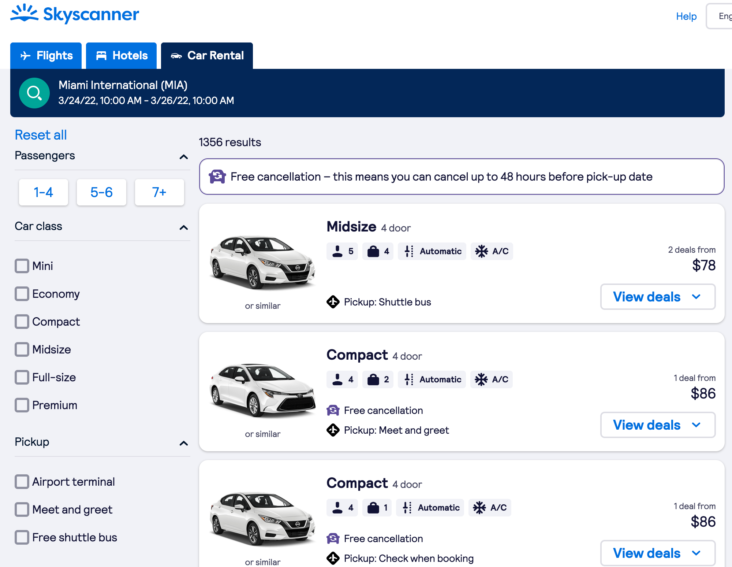The image depicts a booking interface with a gray background and the Sky Scanner logo in blue. At the top of the interface is an image of the sun accompanied by the word "HELP" and options for booking "flights," "hotels," and "car rentals." The term "Carventel" is highlighted in dark blue along with "Miami International (MIA Miami International)."

The travel dates displayed are "03/24/22 10:00 AM to 03/26/22 10:00 AM." A green circle with a magnifying glass icon indicates a search function next to a "reset all passengers" option, which includes dropdown selections for "1 to 4 passengers," "5 to 6 passengers," and "7 plus passengers." Car class options are listed as "mini," "economy," "compact," "mid-size," "full-size," "premium," "pickup," and features like "airport terminal," "meet and greet," and "free shuttle bus" are available. 

There are 1,356 results displayed, and a "free cancellation" note informs users that cancellations are allowed up to 48 hours before the pickup date. Car rental deals listed include a mid-size four-door vehicle available from $78 with two deals, and a compact four-door vehicle available from $86 with one deal.